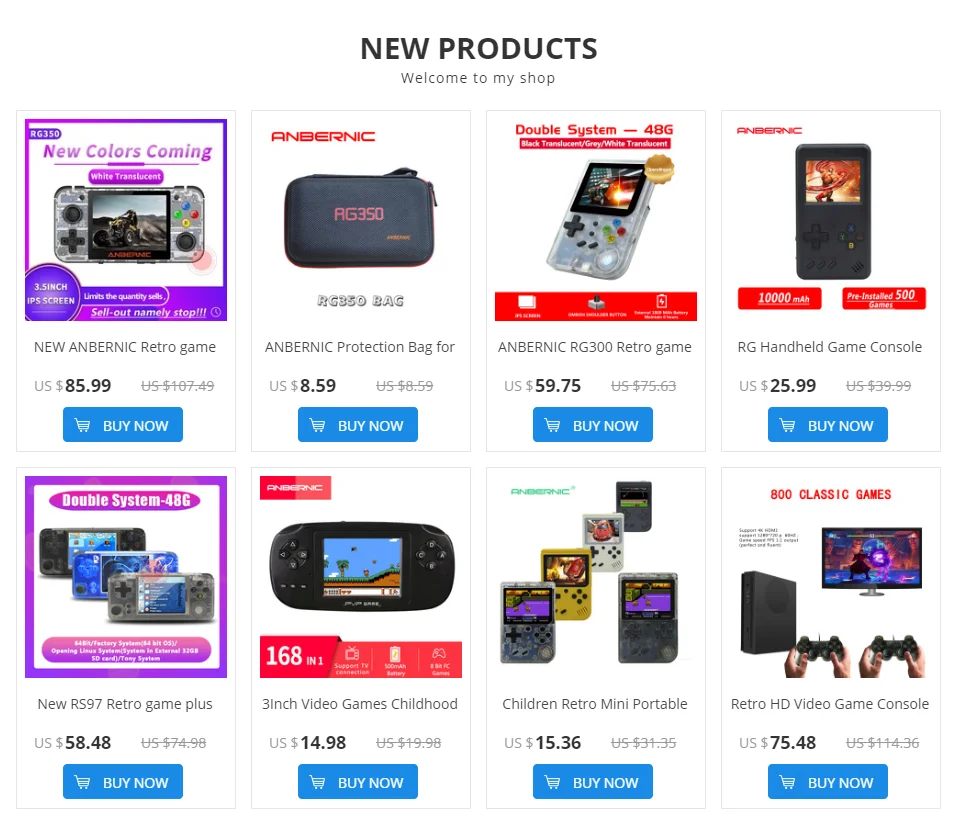Screenshot of an Online Shop Page Featuring New Retro Gaming Products:

This screenshot captures an online store page showcasing a variety of new products, particularly emphasizing retro gaming systems. The seller, likely involved in dropshipping or offering a wide array of products, features several retro game consoles and accessories.

Highlighted products include the "Anbernic Retro Game" console, available in its original white translucent color, with new colors soon to be released. This console boasts a 3.5-inch IPS screen.

Also listed is an Anbernic protection bag designed for the gaming system, ensuring safe transportation and storage. Additionally, the shop offers a double system console available in black, translucent gray, and white translucent variants.

A noteworthy feature is the RG handheld game console, pre-installed with an assortment of nostalgic games. Another product, the new RS-97 retro game console, comes with a 3-inch screen and 168 classic games packaged in one compact system, reminiscent of an old Game Boy.

For those seeking a broader retro experience, the shop provides an 800 classic games retro HD video game console. All these products are currently on sale, with original prices struck through and reduced prices prominently displayed.

Various options are available for immediate purchase, inviting customers to take advantage of the ongoing promotions and clearance deals.